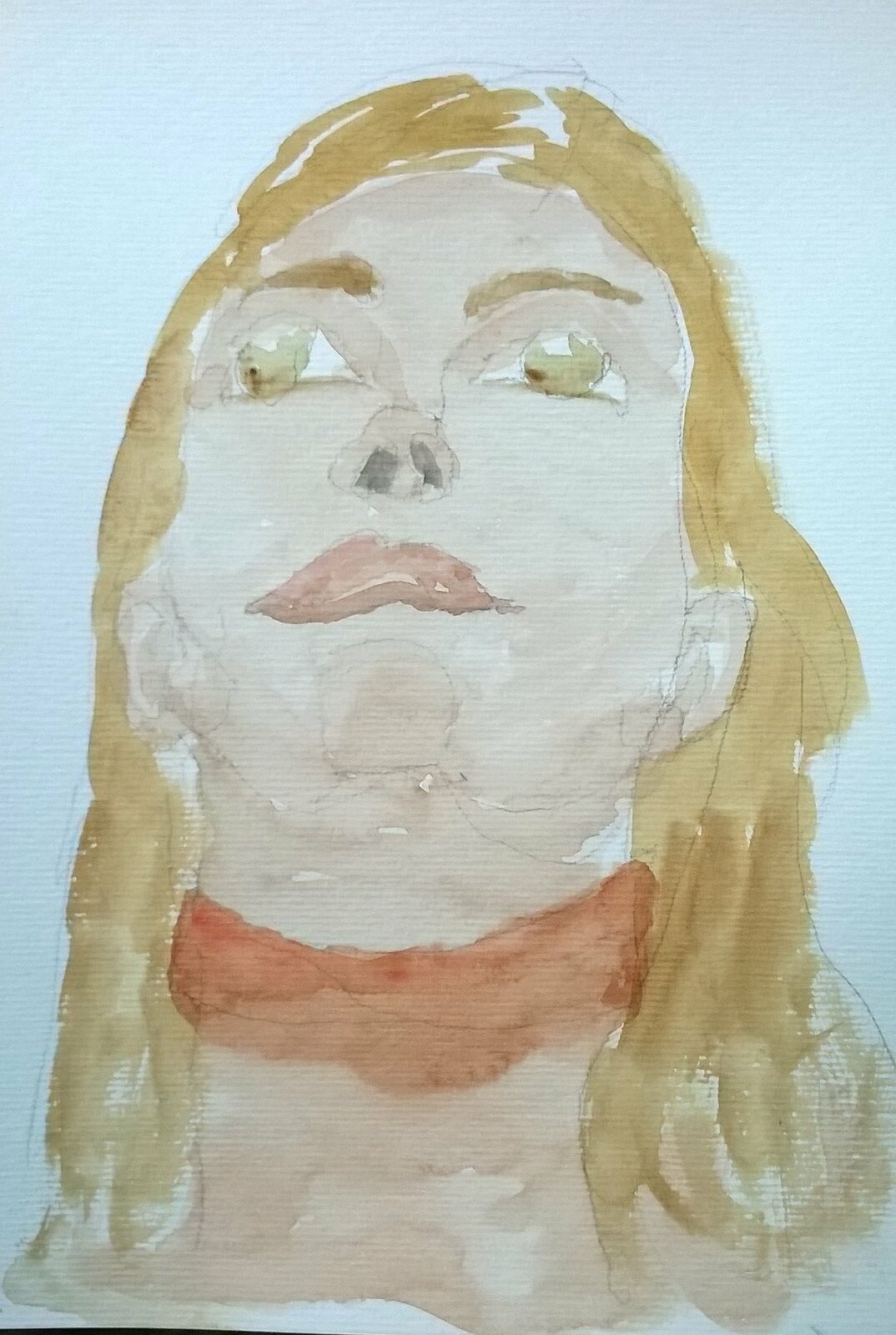This watercolor painting, rendered on white paper, features the portrait of a woman with a pastel-themed palette. The woman gazes upward, her red lips adding a vibrant contrast to the subtle hues. Her shoulder-length hair, in shades of dark blonde or light brown, frames her face, while a striking red band across her neck hints at either a necklace or the top of her garment. Her eyes and eyebrows mirror the hazel tones of her hair, creating a harmonious color scheme. Notably, her ears are positioned unusually low, close to her neck, adding a distinctive characteristic to the artwork. The composition focuses solely on her head and neck, making it an intimate and captivating portrayal.